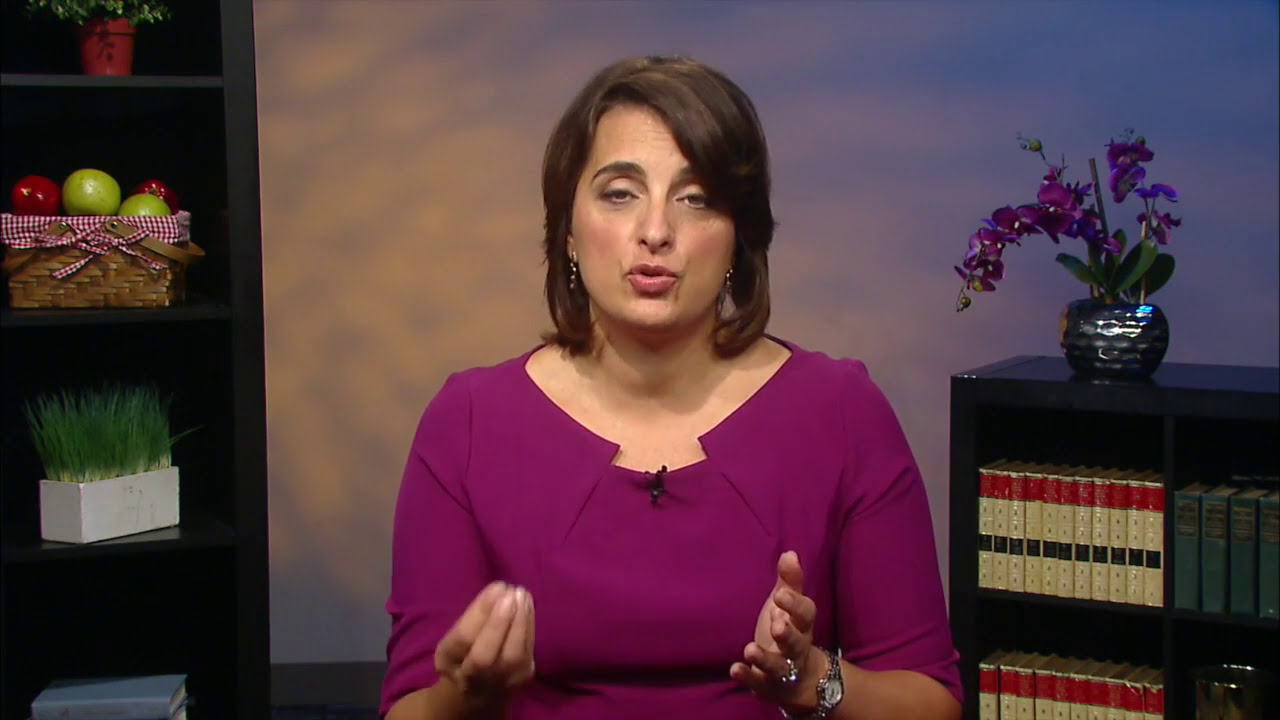In the image, we see a woman with brown hair that is neck-length, styled with short, silver-looking earrings, and a wristwatch. She's wearing a magenta or dark purple top and has her hands extended towards the camera, suggesting she might be explaining something. Her expression includes puckered lips as if mid-sentence, and her eyes are partially lidded.

The background features an indoor setting with two bookshelves. To the bottom right of the image, a black bookshelf holds a flowerpot with purple orchids, adorned with green leaves, and a small green plant below. Off to the left, a higher black bookshelf is seen containing a straw basket filled with shiny red and green apples and another basket with fake grass. 

The photograph does not contain any text or words. The visible colors include fuchsia, tan, red, light green, dark red, light purple, and silver. Although the image cuts off at her waist, it is unclear if the woman is sitting or standing. The scene appears to be staged indoors and resembles a setting akin to a TV show.